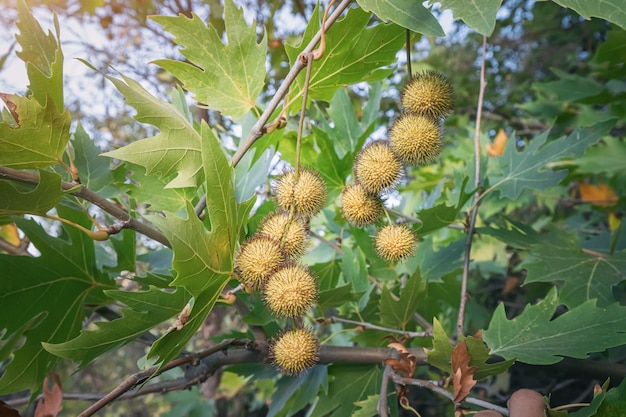This detailed photograph captures a close-up of a tree branch adorned with clusters of small, spherical yellow fruits, each encased in numerous brown, spiky protrusions. The vibrant green leaves of the tree, shaped like three-fingered tips with prominent veins displayed in a light golden hue similar to the fruits, form a striking contrast against the pale blue sky in the blurred background. These leaves show a dual-toned color—a vivid green on the top and a pale yellow on the underside. Interspersed among the foliage, the sunlight filters through, highlighting the natural textures and creating an interplay of light and shadow. The scene is completed with additional branches and leaves tinged with yellow and brown, emphasizing the outdoor, nature-filled setting.